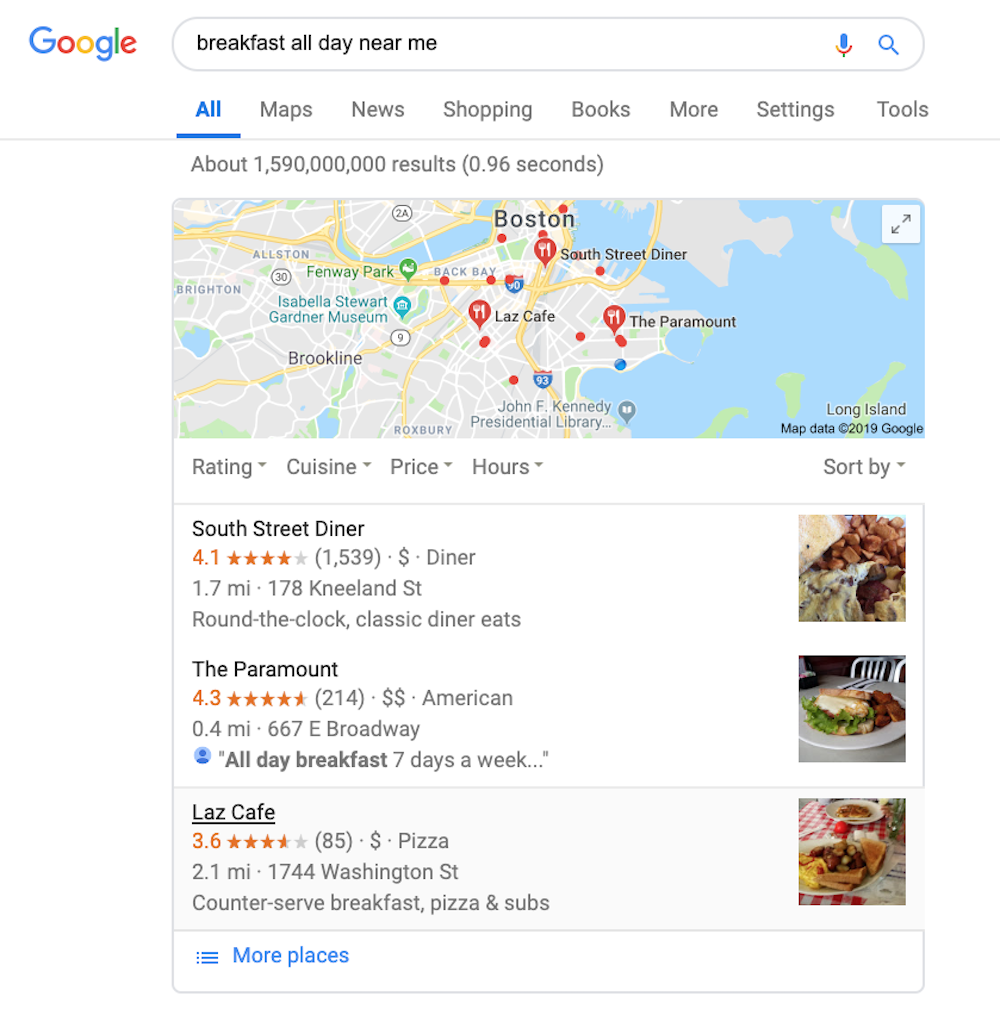In this image, we see a detailed search result for "breakfast all day near me." The search engine has provided approximately 1,590,000,000 results in just 0.96 seconds. The screen features various tabs including Maps, News, Shopping, Books, Mall, Settings, and Tools.

A map is prominently displayed, showcasing several locations related to the search. Key points of interest marked on the map include Boston, Brooklyn, Long Island, and Roxbury. Specific landmarks noted are the South Street Diner, The Paramount, and Last Cafe, as well as the Isabella Stewart Gardner Museum, Fenway Park, and the John F. Kennedy Presidential Library.

Detailed ratings and reviews accompany the featured breakfast spots:
- South Street Diner: 4.1 stars from 1,539 reviews
- The Paramount: 4.3 stars from 214 reviews
- Last Cafe: 3.6 stars from 85 reviews

These ratings provide insight into the popularity and reputation of the dining establishments, aiding users in making informed choices for an all-day breakfast option.